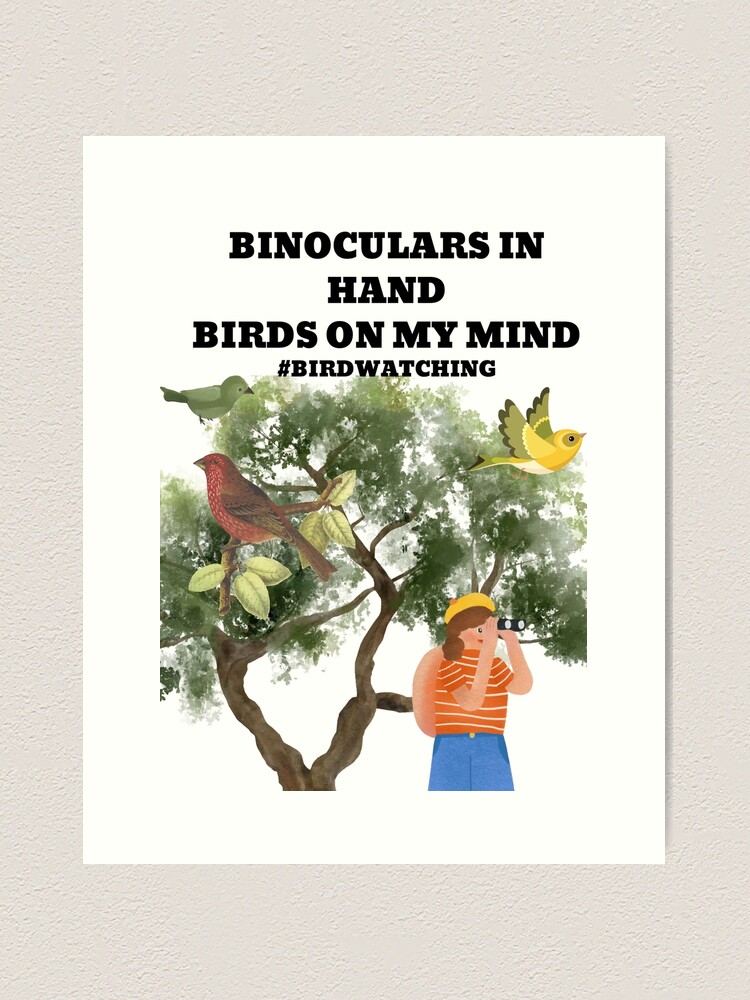A white poster is affixed to a pristine white wall, creating a seamless and minimalist aesthetic. At the top of the poster, bold black lettering prominently declares, "Binoculars in hand, birds on my mind," capturing the essence of the subject's passion for bird watching. Beneath this phrase, a smaller line of text features a hashtag, "#birdwatching," cementing its theme and engaging an online audience. Dominating the majority of the poster is an intricate illustration of a tree, its branches home to three birds. In the bottom right corner, a figure stands facing right, intently peering through binoculars, fully immersed in observing the avian world above.